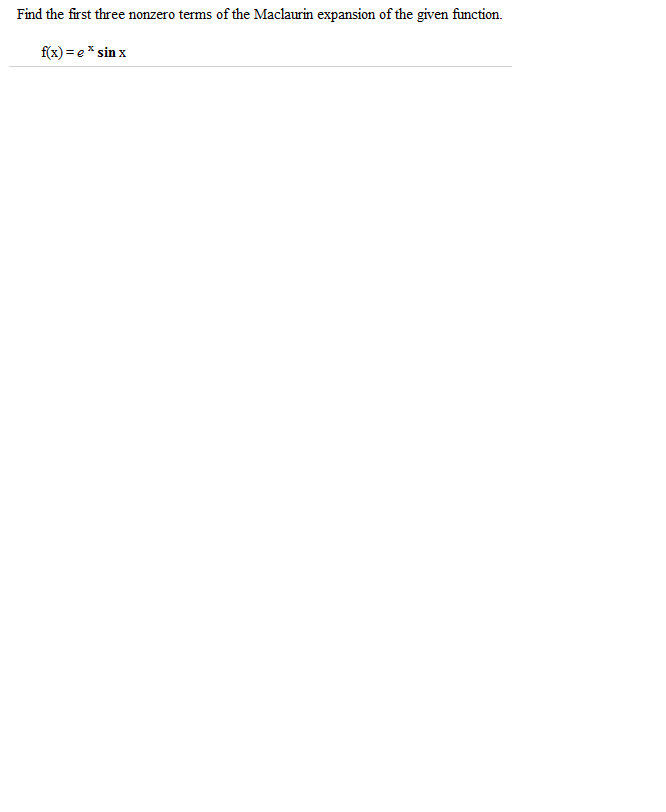A minimalistic and straightforward image set against a white background. At the top, there is a simple black sentence stating: "I'll find the first three nonzero terms of the Maclaurin expansion of the given function." Below this sentence, slightly indented, the mathematical expression is presented, reading: "F(x) = e^x * sin(x)." The overall appearance suggests that the content might be notes or a prompt for solving a math problem involving the Maclaurin series expansion. The plain and uncluttered nature of the image emphasizes the core focus on the mathematical task at hand.